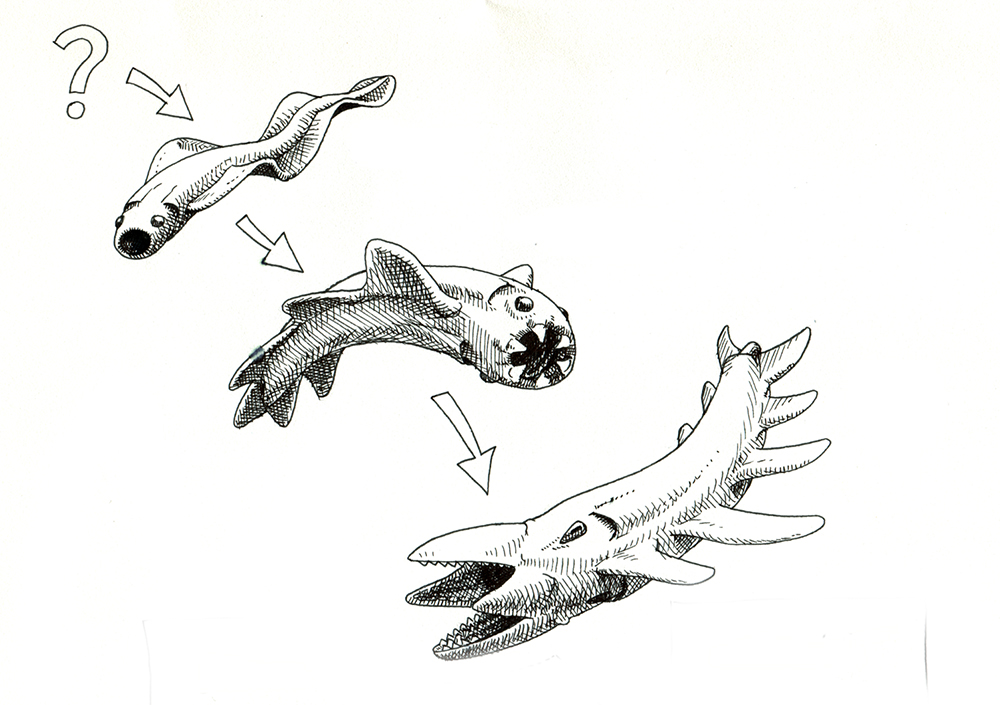This black and white image depicts a detailed, hand-drawn evolutionary sequence of a fictional aquatic creature. In the top right corner, a question mark signals the beginning of the transformation process, linked by an arrow to the initial stage of the creature—a long, tube-shaped fish resembling an eel or tadpole. This early form features two fins that connect to its tail, a flat round mouth, and distinct black eyes. 

From this first stage, an arrow directs down to an intermediate version where notable changes are evident: the fish now has a wavy, elongated fin and displays sharp teeth within its more pronounced mouth. The structure appears shorter and more compact than before.

Continuing the sequence, another arrow points to the final evolved form of the creature. Here, the fish has dramatically transformed—sporting ten individual fins along its body and a mouth that divides into four sections. This ultimate form also has numerous, smaller sharp teeth, enhancing its monstrous appearance. Each evolutionary stage is meticulously rendered, highlighting the gradual yet significant anatomical transformations from a primitive eel-like fish to a more complex, alien-like entity, reminiscent of creatures from science fiction narratives such as Stranger Things.